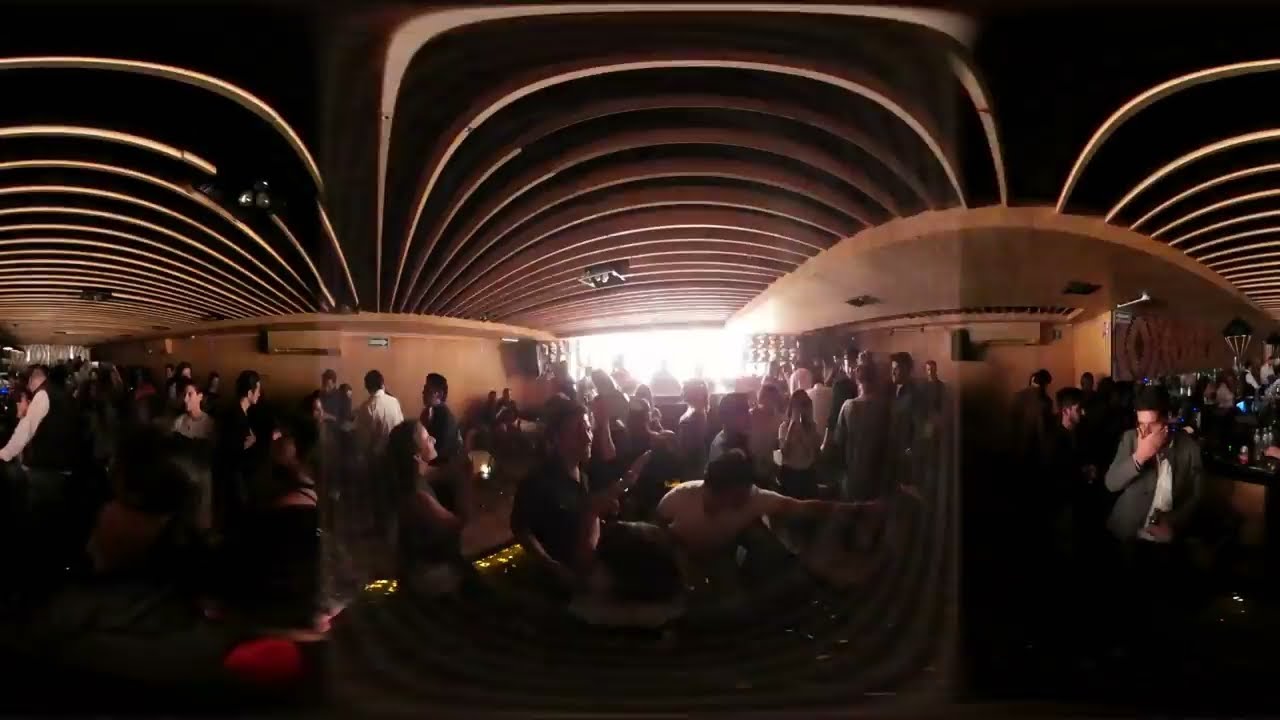The image captures a dimly lit, crowded interior of a modern, possibly futuristic building. The ceiling, painted black, features brown, curved architectural shapes that give a stylish, modern flair to the space. A tan, curved wooden wall dominates the scene along with curved wood beams on the ceiling. The entrance, illuminated with light, is visible straight ahead.

Amidst this setting, a multitude of people fill the room, their activities obscured by the dim lighting. They appear to be standing around, engaging in conversation, taking pictures, and looking up. Among the crowd, key details emerge: a person in the foreground wears a long-sleeved jacket with a white shirt underneath, and another individual on the far left dons a waiter's outfit, characterized by a long white shirt and a black vest. Additionally, there seems to be someone holding an indistinct instrument, possibly a guitar, adding a layer of ambiguity to the bustling yet unclear atmosphere. The overall scene suggests the gathering could be taking place in a restaurant, bar, or similar venue.